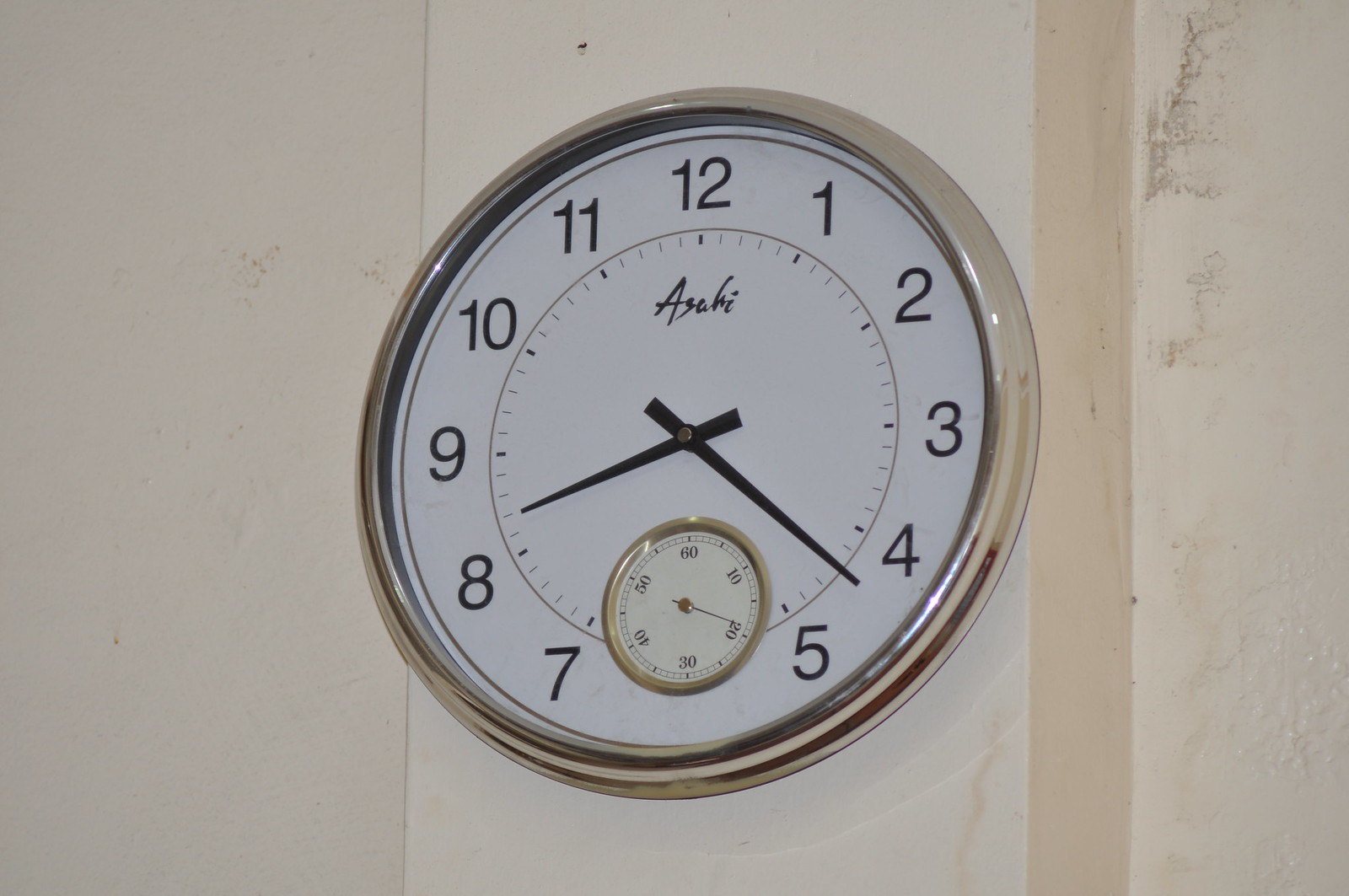This photograph features a simple, round wall clock encased in a sleek silver frame, showcasing a clean white face with prominently displayed black Arabic numerals. The characters read 1 through 12, except for the number '6,' which is conspicuously absent. The brand name "Asahi" is inscribed above the two black hands, which indicate a time of 8:22. Enhancing its functionality, the clock also includes a barometer inset into its face. This barometer section is in a slightly darker shade of white, encircled by a brass ring. The clock is mounted on a wall painted in a somewhat grimy beige-peach hue, adding a rustic backdrop to the polished timepiece.